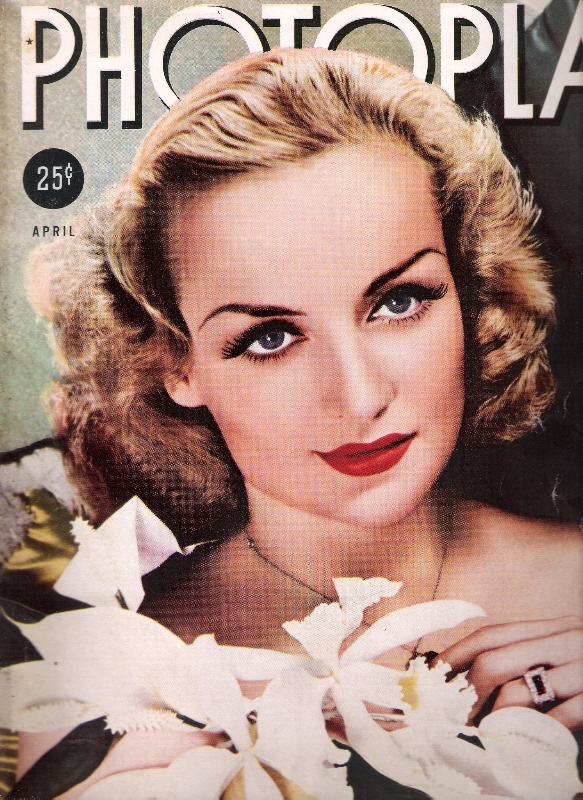The image depicts an old-fashioned magazine cover, likely from a publication titled "Photoplay" though the full name is partially cut off after "photo." The cover features a blonde woman with shoulder-length, curly hair styled in a classic cinematic fashion. Her makeup is distinct with red lipstick, mascara, and grey or blue eyes. She appears to be holding a bouquet of white flowers in front of her chest, possibly obscuring her clothing. Notably, she is also wearing a ring and a necklace, which she seems to be pinching with her left hand. In the top left corner of the cover, a black circle contains the price of 25 cents in white text, indicative of the magazine's age. Below the price, the word "April" is printed in small black text. The overall quality of the image suggests it has been around for many years.